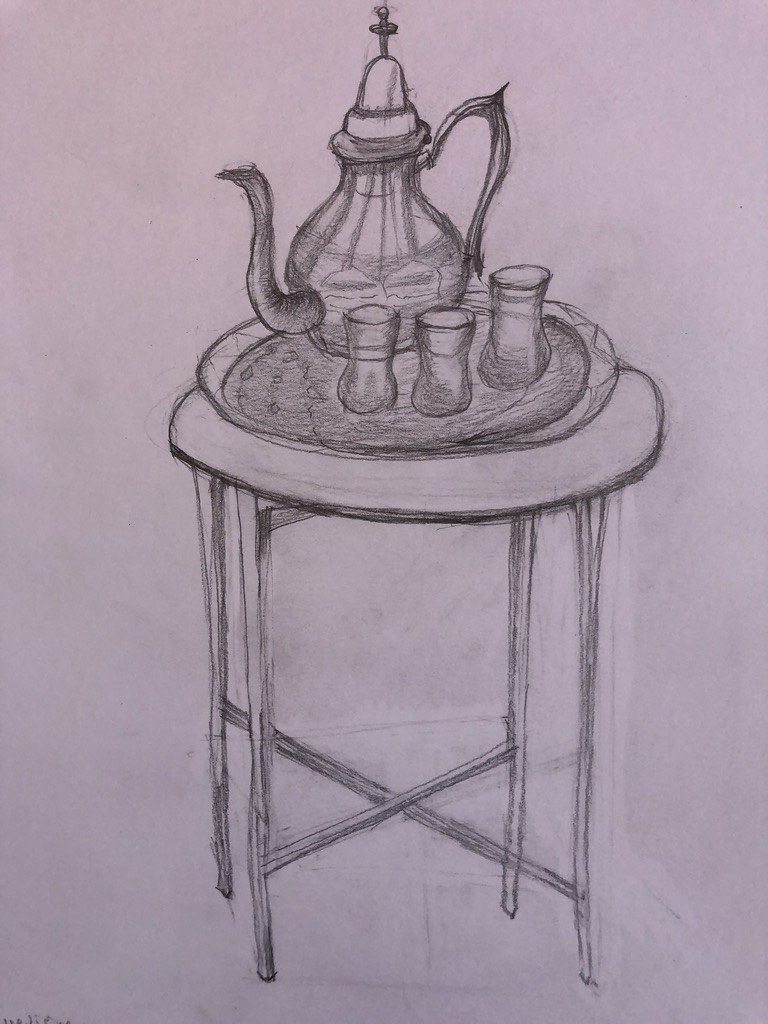A meticulously detailed pencil drawing on a light lavender-colored paper showcases a circular end table with four gracefully extending legs. The legs are reinforced by crossed support beams at the bottom, adding structural stability. Subtle erasure marks are visible around the legs, revealing the artist's process. Atop the table, a well-shaded gray platter is neatly arranged with three glasses and a tea kettle. The tea kettle, capped with a pointed cross lid, adds a touch of elegance to the tranquil scene.